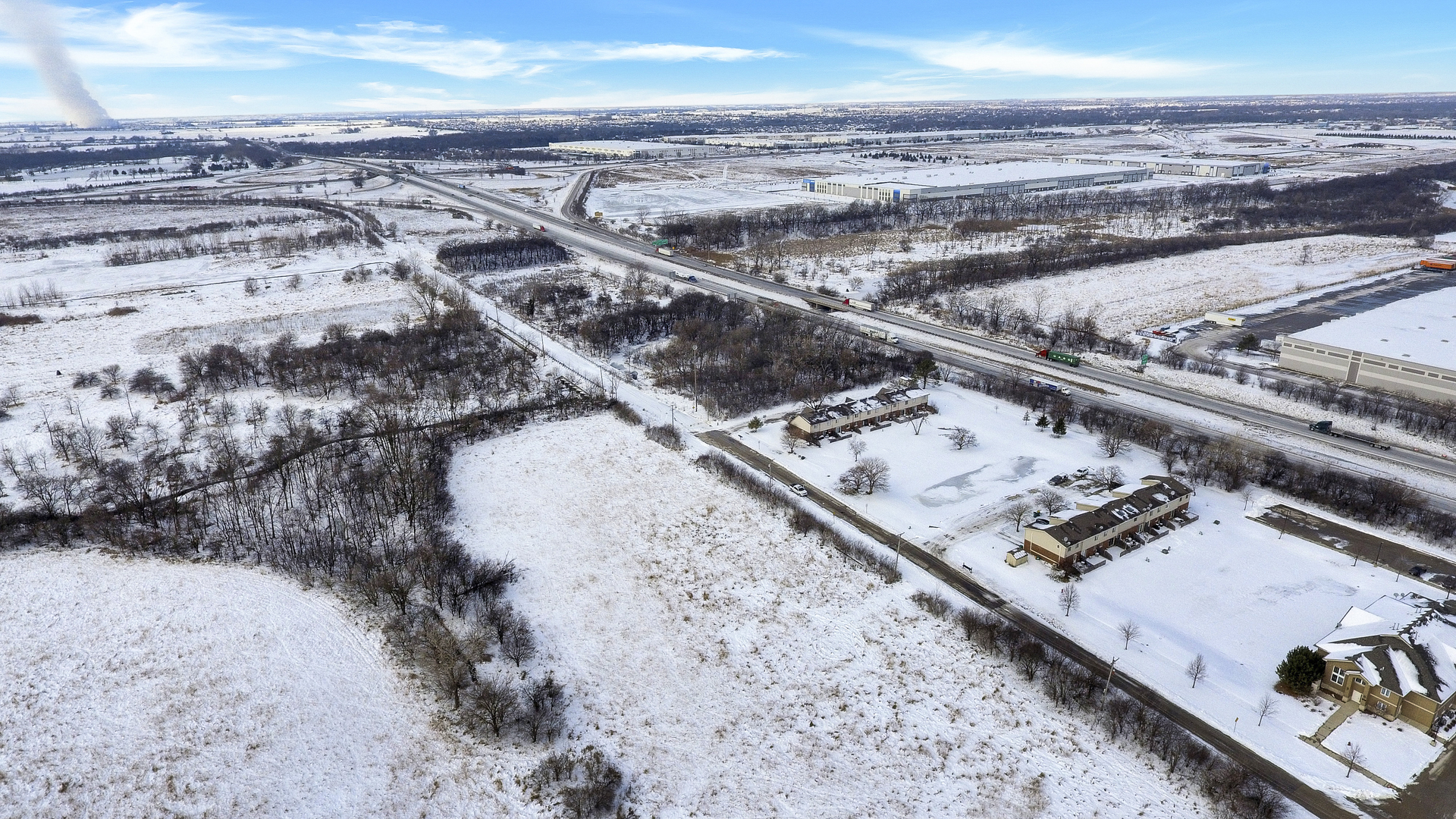This image is an aerial view of a rural town captured from a helicopter. The landscape is predominantly covered in snow, creating a stark white backdrop dotted with dormant winter trees. The sky is clear and blue, with a few wispy clouds hinting at the cold winter day. Two major roads run prominently across the scene, and nestled between them are three distinct buildings. The first building appears to be a residence, with a single walkway and snow-covered roof. The middle building, believed to be a motel or office due to the number of cars parked around it, occupies more space. The third structure, likely an outbuilding or office, stands isolated without obvious walkways or plowing around it. Despite the serene winter landscape, a dramatic and concerning feature dominates the top left corner—a tiny yet formidable tornado funnel looms menacingly, poised to ravage the roads and vehicles in its path. The vast expanse of the town reveals an otherwise flat and open terrain, with patches of trees and sprawling snowy fields extending into the horizon.